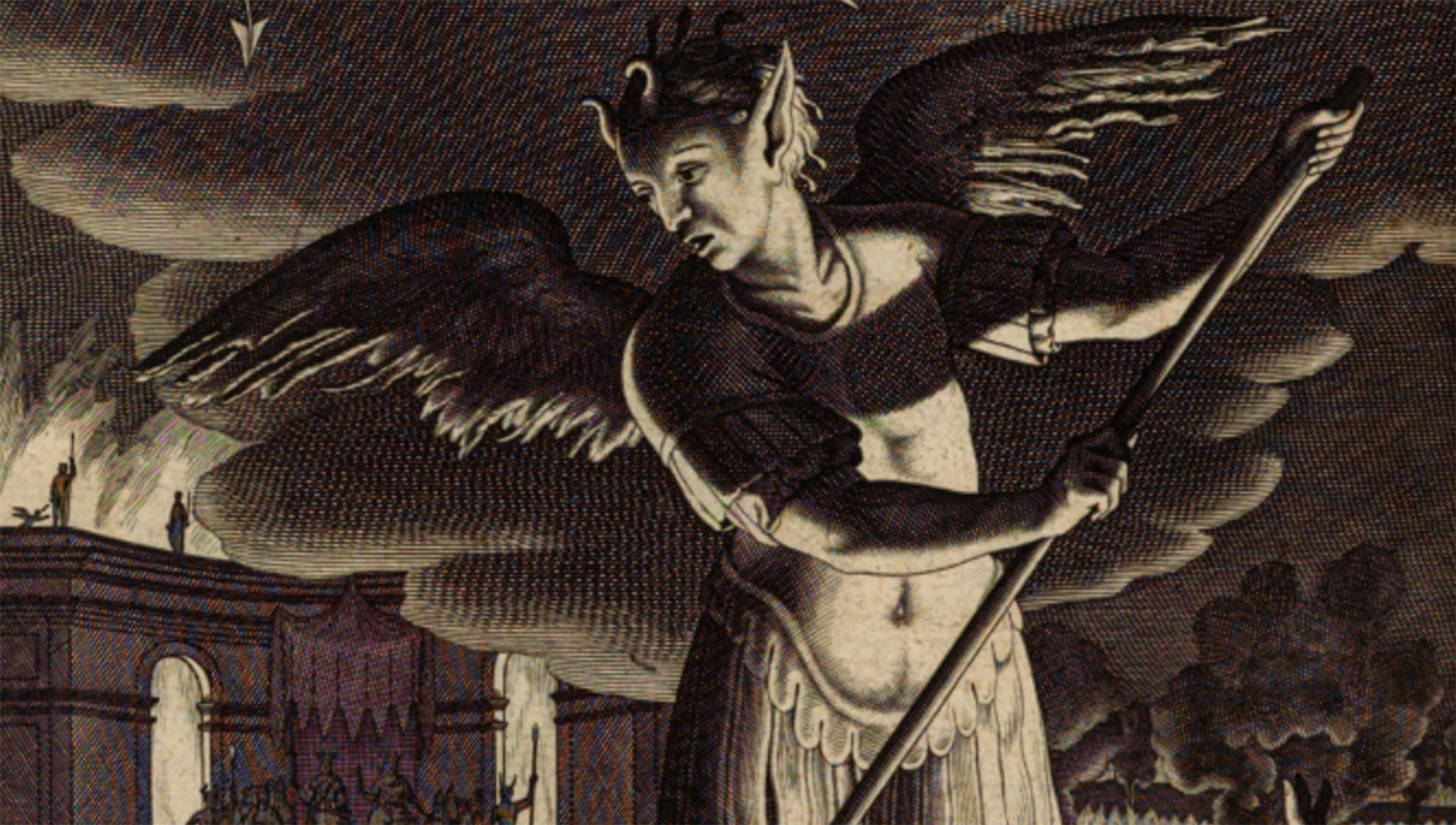This intricate black-and-white sketch from the 1930s or 1940s showcases a mythological scene with a strong and dark atmosphere. At its center is a human-shaped creature resembling an angel, complete with large, curvy wings and long, pointy ears, topped with a tuft of fur-like detail. The figure gazes towards the bottom left corner, holding a wooden pole or broomstick. The background reveals a complex arrangement of buildings featuring arched gates, with soldiers holding spears standing on and around them. Dark clouds and trees, which resemble vegetables, add to the somber mood of the illustration. The bottom right hints at a dense forest while the bottom left features a significant fire. The overall complexity, full of shapes and patterns, encapsulates the essence of an elaborate mythological artwork.